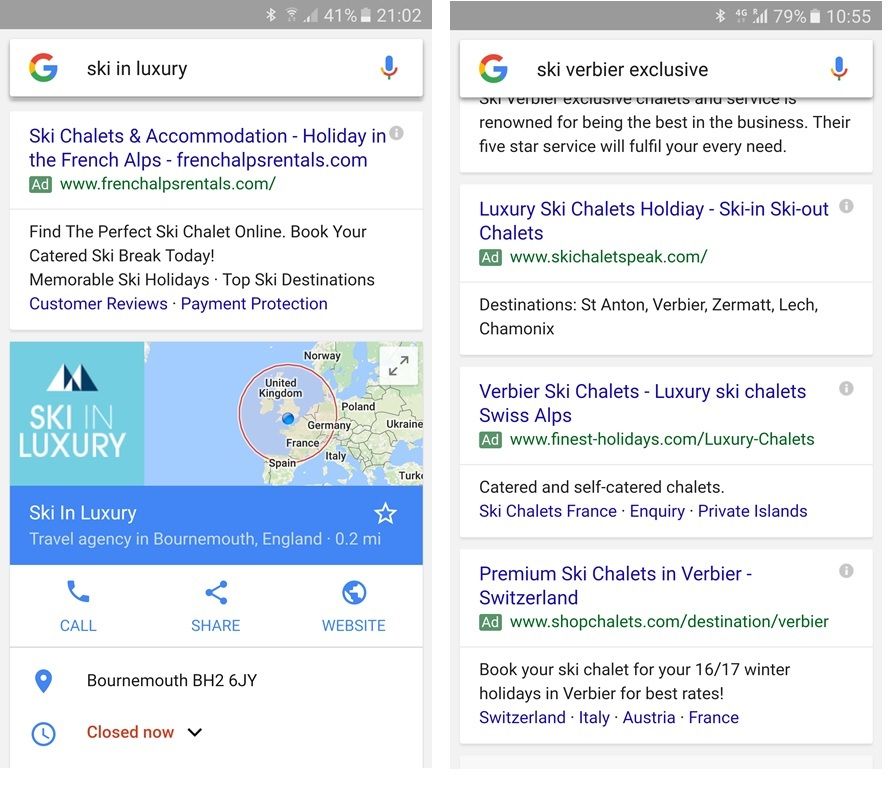The image depicts two screens positioned side by side. 

On the left screen, various interface elements are displayed. In the upper right corner, a series of icons are seen in the following sequence from left to right: a Bluetooth icon, a Wi-Fi icon, a cellular signal icon. Additionally, a percentage figure "41%" appears next to a battery icon, and the time is denoted as "21:02".

Directly below these icons, there is a search bar. On the left side of this search bar, the Google logo, represented by a stylized "G", is visible. The search query entered into the bar reads "ski in luxury." On the far right inside the search bar, there is a microphone icon.

Further down, textual information reads "ski chalet and accommodation - holiday in the French Alps - FrenchAlpsRentals.com." Note that "chalet" is misspelled as "C-H-A-L-E-S-T-S" and "Alps" is misspelled as "L-A-P-S".

The right screen remains unspecified in the description, omitting any details about its contents or purpose.